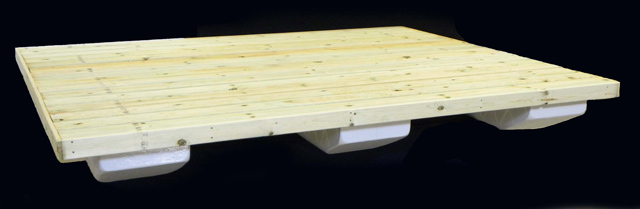The image showcases a smooth, rectangular wooden board with a light yellow to cream color gradient, featuring scattered darker gray speckles and dots. The board rests on a white, flat base, supported by three white structural elements evenly spaced from left to right. This entire setup is placed against a completely black background, emphasizing the contrasting colors and textures of the board and its supports. The solid black backdrop lacks any additional graphics or designs, highlighting the distinct details of the board and its foundational elements.